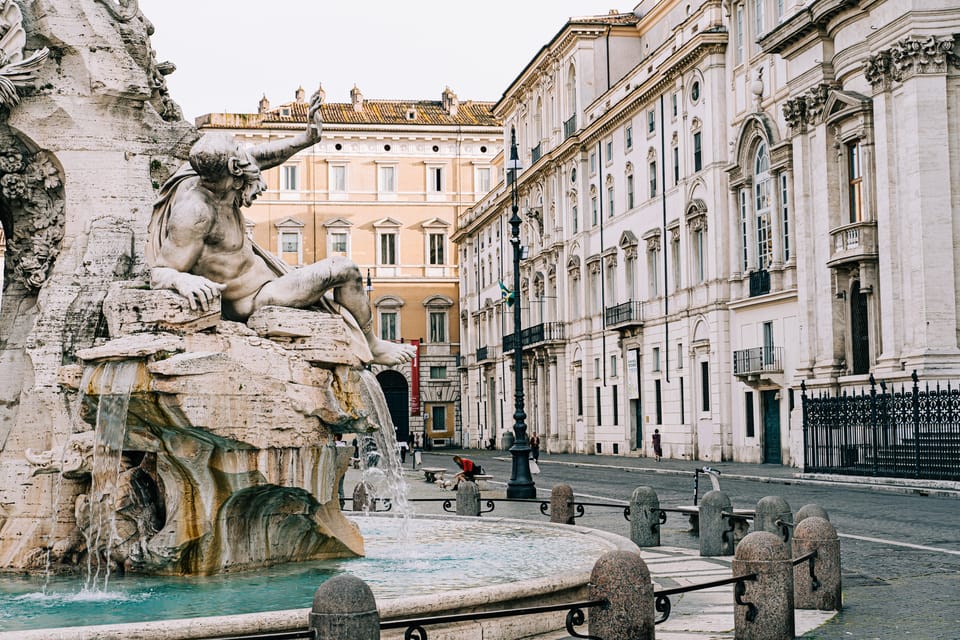In this photo of a European town square, a prominent and very elegant fountain is situated on the left side. The fountain features a detailed sculpture of an older bearded man with a bald head, sitting on rocks. He has his right leg crossed over his left and is propping himself up with his right arm while his left arm is held up, as if blocking something. The man is draped in a material across his body, otherwise unclothed. Clear, bluish or greenish water flows from the rocks beneath him into the base of the fountain, which is surrounded by a shin-high fence made of stones interspersed with cast iron.

On the right side of the image, there are large, old buildings showcasing European-style architecture, tan-colored and distinguished in appearance, possibly government buildings. In front of these buildings, a street stretches out, devoid of cars. A person in a red shirt is sitting on a bench with a dog in front of her, while two other people walk on the sidewalk. In the background, there is a large, orange-ish, peach-colored building with a brownish roof, which appears to be an apartment complex. The scene is serene and captures the essence of a historical European town square.